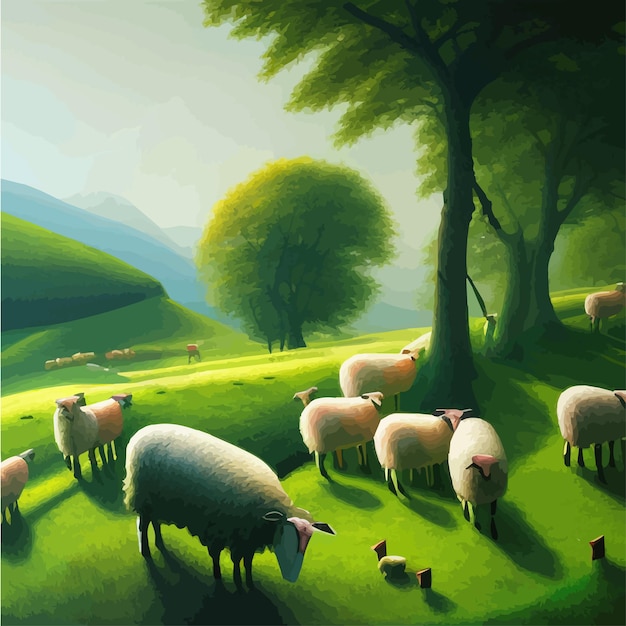This digitally created square artwork portrays a vibrant outdoor scene with a group of chunky, round, and fluffy sheep grazing on bright green, rolling hills. The sheep, predominantly gathered in the lower right foreground, sport an off-white hue that accentuates their well-fed appearance. The hilly meadow is dotted with trees, some with bright green treetops, particularly on the right side of the image. The landscape descends into a valley towards the middle, where a large round tree stands prominently. Farther back, the terrain rises again, leading to distant mountains. The sky at the top left of the picture is a cloudy white, enhancing the overall bright and cheerful daytime setting. Scattered throughout are subtle hues of light green, light yellow, dark green, tan, beige, and black, contributing to the rich, idyllic countryside atmosphere.